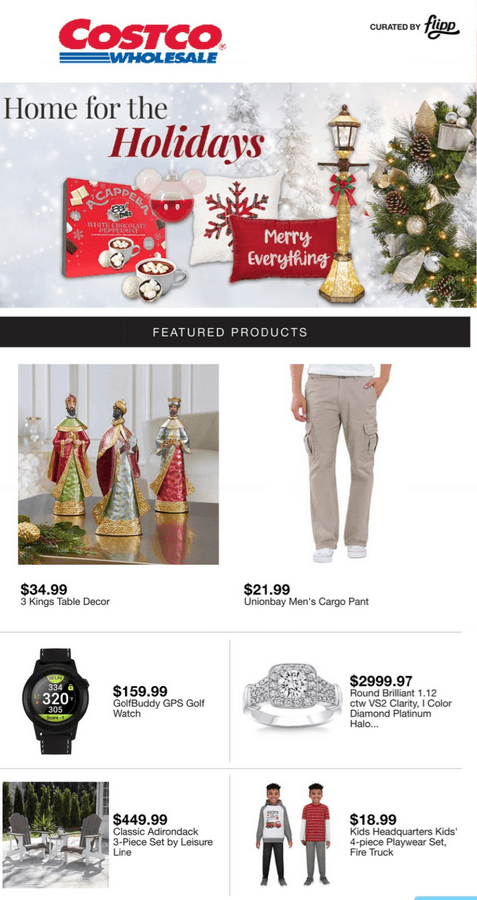This image showcases a Costco website layout. At the top, the traditional Costco logo in red is prominently displayed, accompanied by the word "wholesale" in blue, stylized with three motion lines. To the right, the text "curated by Flip" is featured, with "Flip" partially written in cursive.

Beneath this header, there is a holiday-themed banner with the message "Home for the Holidays" where "Holidays" is italicized and colored red. Below the banner, there are images of festive items including a "Merry Everything" pillow, a pillow with a snowflake design, a lamp stand to the right, and a hot chocolate setup on the left.

A black banner titled "Featured Products" divides the section below, showcasing various items for sale. Listed products include:

- A Three Kings table decor for $34.99.
- A pair of brown pants for $21.99 worn by a model.
- A Golf Buddy GPS for $159.
- A ring priced at $2,999.97.
- Children's attire for $18.99.
- A classic three-piece outdoor leisure set on the left for $449.

Each product is accompanied by its price, offering a detailed glimpse into Costco's holiday-season promotions.